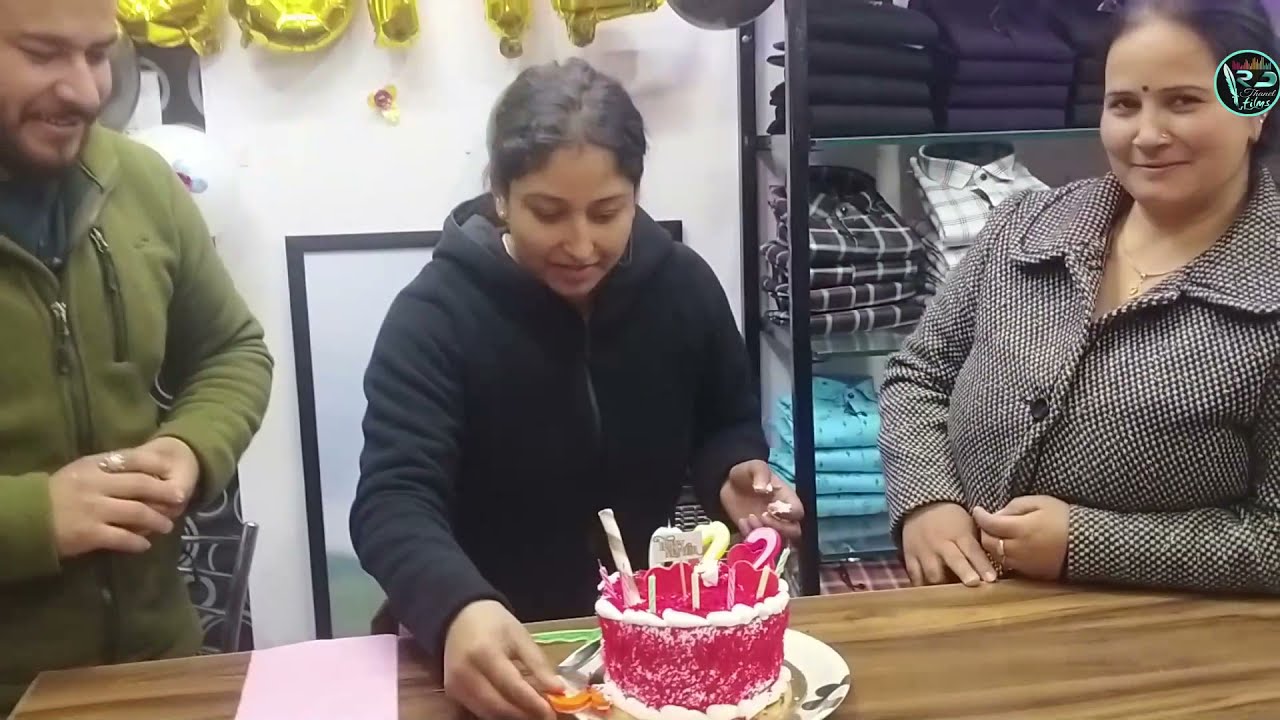In this celebratory birthday photograph, three people are gathered around a wooden table adorned with a festively decorated cake. The central figure is a young, dark-haired woman, seemingly in her late teens, with her hair pulled back. She is dressed in a black hoodie and is leaning over the cake, smiling and appearing to place or grab something from it. The cake, positioned on a silver platter, features red icing with white frosting trim and is topped with candles and candies. 

To her left, on the right side of the photograph, stands a middle-aged woman with a warm smile, wearing a checkered black-and-white jacket and a necklace. Behind her, labeled displays of stacked shirts suggest they are in a store setting. To the young woman’s right, on the left side of the image, is a bearded man in a green fleece jacket, smiling down at the cake. Both adults may be the young woman's parents.

The backdrop includes a white wall adorned with gold balloons on the left and a circular logo in the upper right corner, partially obscured. This well-lit scene captures the joy and warmth of a familial birthday celebration within what appears to be a retail setting.